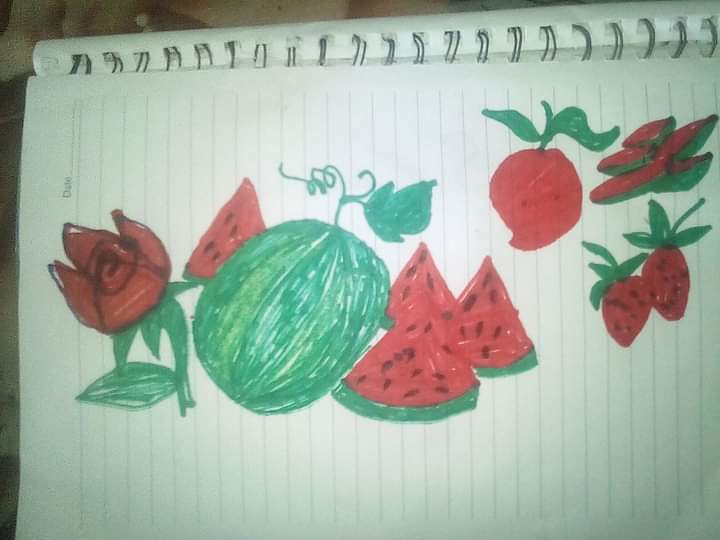This top-down photograph of a horizontally-laid spiral-bound lined notebook captures a detailed, hand-drawn illustration done primarily in red, green, and black markers. The notebook's black metal spiral rings run along the top of the image. On the left side of the page, there's a vibrant red rose with a green stem and a single leaf. Adjacent to the rose, there is a full green watermelon with a squiggly stem and a single leaf, leaning slightly to the right. Four triangular watermelon slices, with green rinds and red flesh dotted with black seeds, are positioned around the whole watermelon—three on the right and one behind it. To the right of these watermelon slices, there are three strawberries: a larger one at the top right, mostly red with a green stem and two leaves, and two smaller strawberries beneath it, both red with green stems and black seeds. The drawing is meticulously detailed, with black outlines accentuating the petals of the rose, the seeds of the watermelon, and the specks on the strawberries.